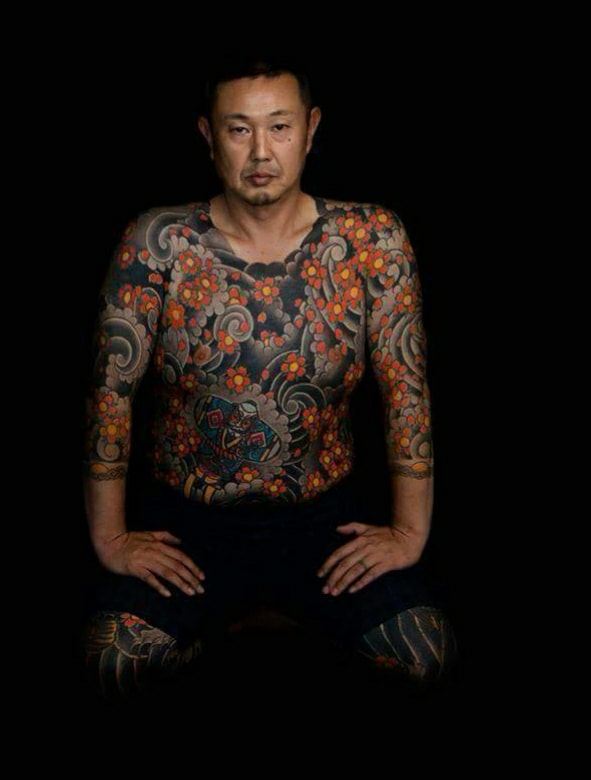The image depicts an East Asian man, possibly of Japanese descent, sitting in a featureless black room with his hands placed inwardly on his upper thighs. His expression is neutral or forlorn, with a slightly closed mouth and short black hair that reveals a bit of his forehead glistening from the light source. The man is wearing only black shorts, exposing his heavily tattooed body. The tattoos consist of dark blue waves or spirals accented with red flowers and yellow centers, reminiscent of poppy flowers. These ornate designs cover his entire torso, shoulders, arms up to his wrists, and his legs, leaving only his neck, hands, and parts of his face untattooed. Notably, his tattoos include a stylized figure, possibly a deity or a religious icon, situated on the lower part of his chest.